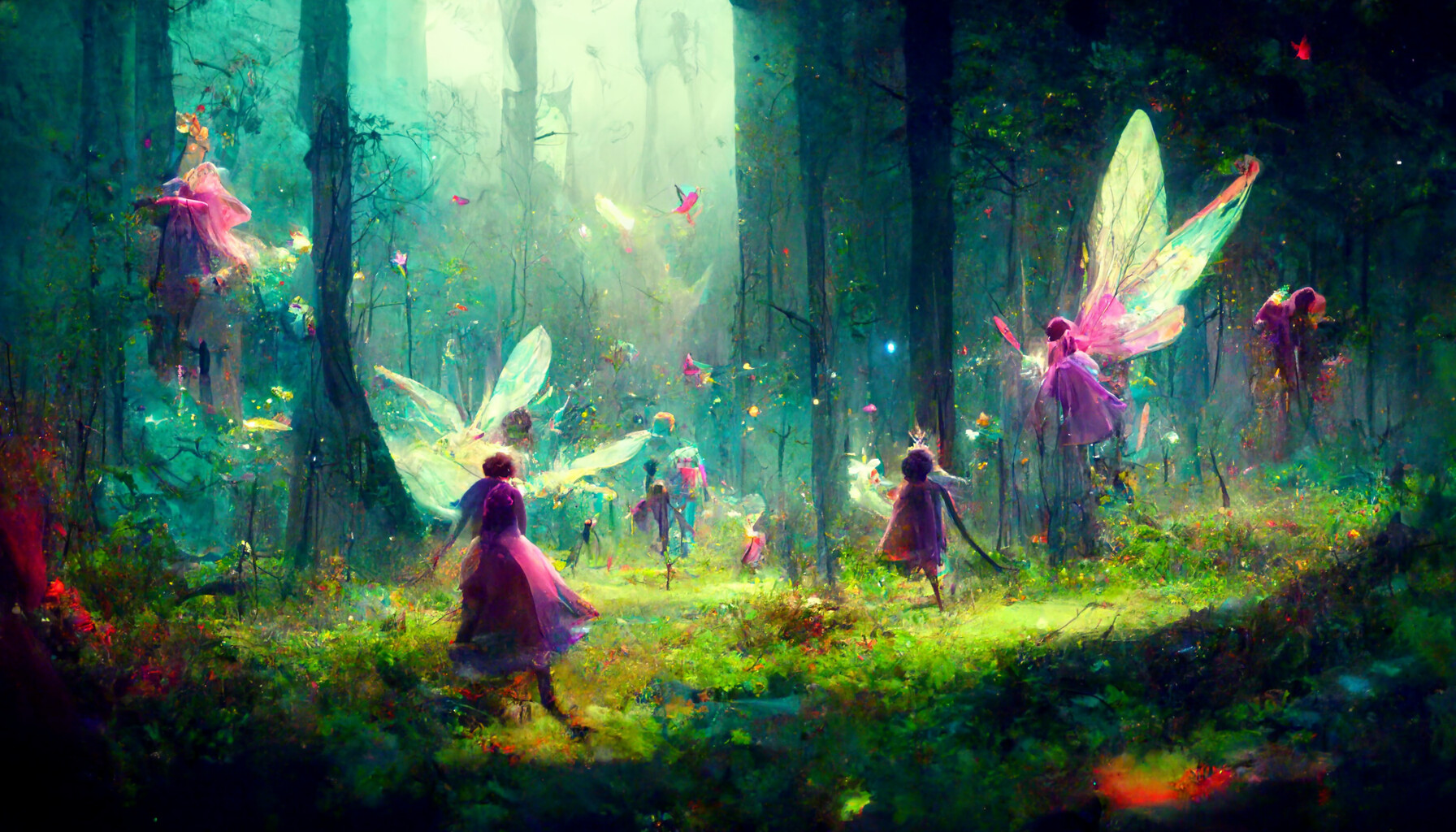The image is a detailed digital depiction that combines elements of a painting and a storybook scene, illustrating an enchanted forest teeming with fairies. Set against a backdrop of tall trees and lush vegetation, various fairies are scattered throughout a grassy field and amongst abundant flowers in the foreground. The image has a dynamic range of light, with shaded dark areas under the treetops transitioning into bright regions illuminated by sunlight filtering through the canopy.

The fairies, predominantly dressed in flowing pink, purple, and lilac gowns, exhibit delicate, almost transparent wings that vary in color from light green to intricate rainbow patterns. There are six prominently visible fairies in the foreground, each appear absorbed in their own activities, while numerous smaller, distant fairies are discernible further back in the forest. The overall color palette of the scene includes shades of green, pink, purple, red, yellow, gold, black, and gray, lending a magical and vibrant atmosphere to the enchanted woodland setting. The image is devoid of any visible text, allowing the viewer to fully immerse in the visual narrative of the fairies’ realm.